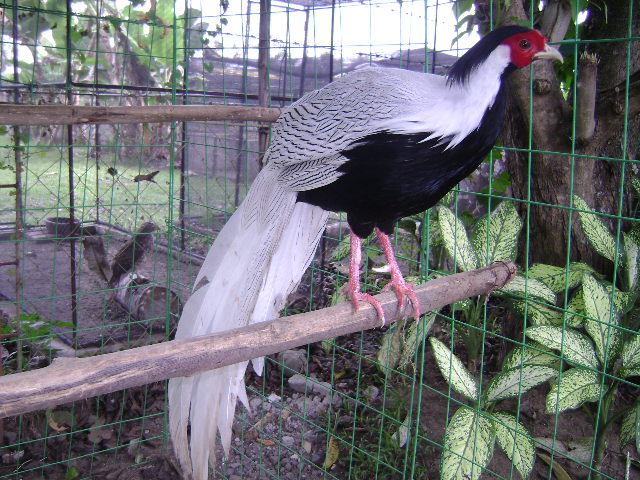This detailed photo showcases a distinctive bird perched on a long tree branch inside an enclosed, green cage. The bird features a strikingly red face with black eyes, a black-feathered top of the head, and a tan-white beak. Its neck is adorned with white feathers, and its body transitions from a white upper part to a black underside. The bird's long, elegant tail feathers are predominantly white, and it stands on pink legs with whitish claws. Surrounding the bird, the enclosure contains green foliage, trees, and shrubbery, with a dirt floor and grass visible in the background. Other birds can be spotted on the ground within the same cage, and a building appears in the background, suggesting this could be a farm, ranch, or large backyard, photographed during daylight.